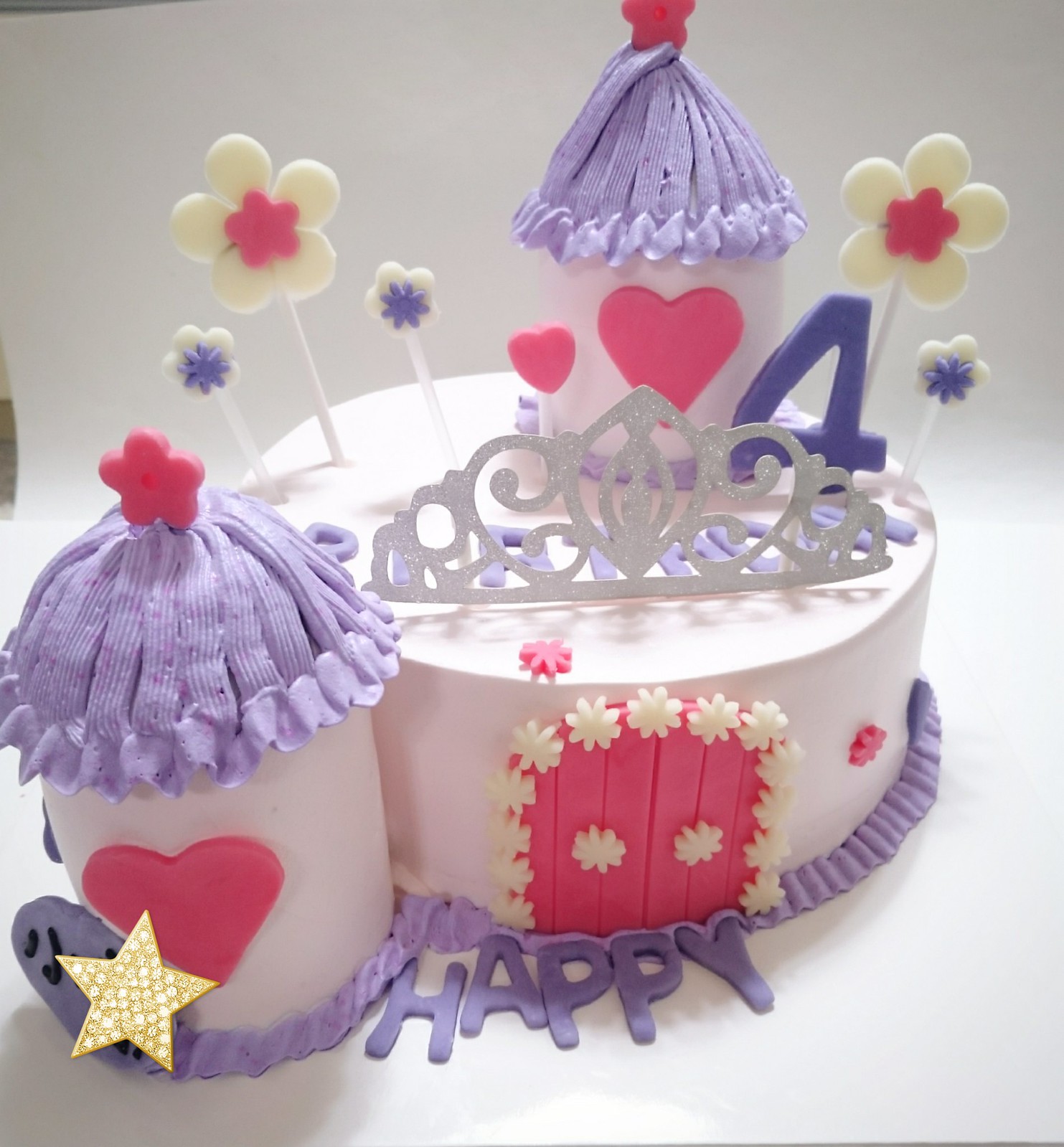This is an image of a detailed birthday cake, celebrating a fourth birthday. The cake itself is mostly white with subtle lavender undertones and adorned with purple frosting piped around the bottom. The front of the cake features the word "happy" in purple letters.

On top of the cake, a glittery silver crown and a purple number four stand prominently. Behind the crown, the word "birthday" is inscribed in a lighter purple hue. Sticking out from the top of the cake are various flower-shaped decorations with either red or purple centers.

The cake embodies a castle theme, featuring two cylindrical towers. The left tower is decorated with a pink heart on the front, a crown on top, a lavender roof, and a pink flower with five petals. The main cake has two red doors in the front surrounded by small white flowers. Another, smaller circular tower is situated next to the number four, featuring a gold star at the base, a pink heart, and a red flower on a purple roof.

Adding to the charming appearance are multiple sticks with various sizes and colors of flowers, harmonizing with the cake's pink, purple, and lavender color scheme.